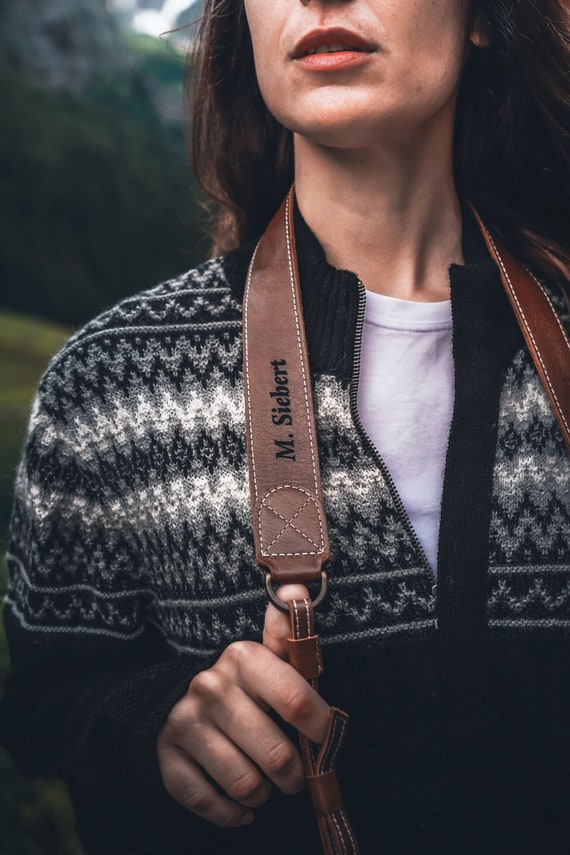The photograph features a young woman, captured from her nose to her midsection, gazing to her right. She has long, dark brown hair flowing past her shoulders and wears striking red lipstick. Her attire consists of a black sweater adorned with intricate white and gray patterns, layered over a white t-shirt. A brown leather strap with the inscription "M. Silbert" drapes around her neck, suggesting it could be for a camera or a bag, which she holds with her right hand. The blurred background showcases a daytime outdoor setting with hints of a mountain, green fields, and trees under a white sky, adding a serene yet dynamic backdrop to the high-definition image, possibly serving as a fashion advertisement or product promotion.